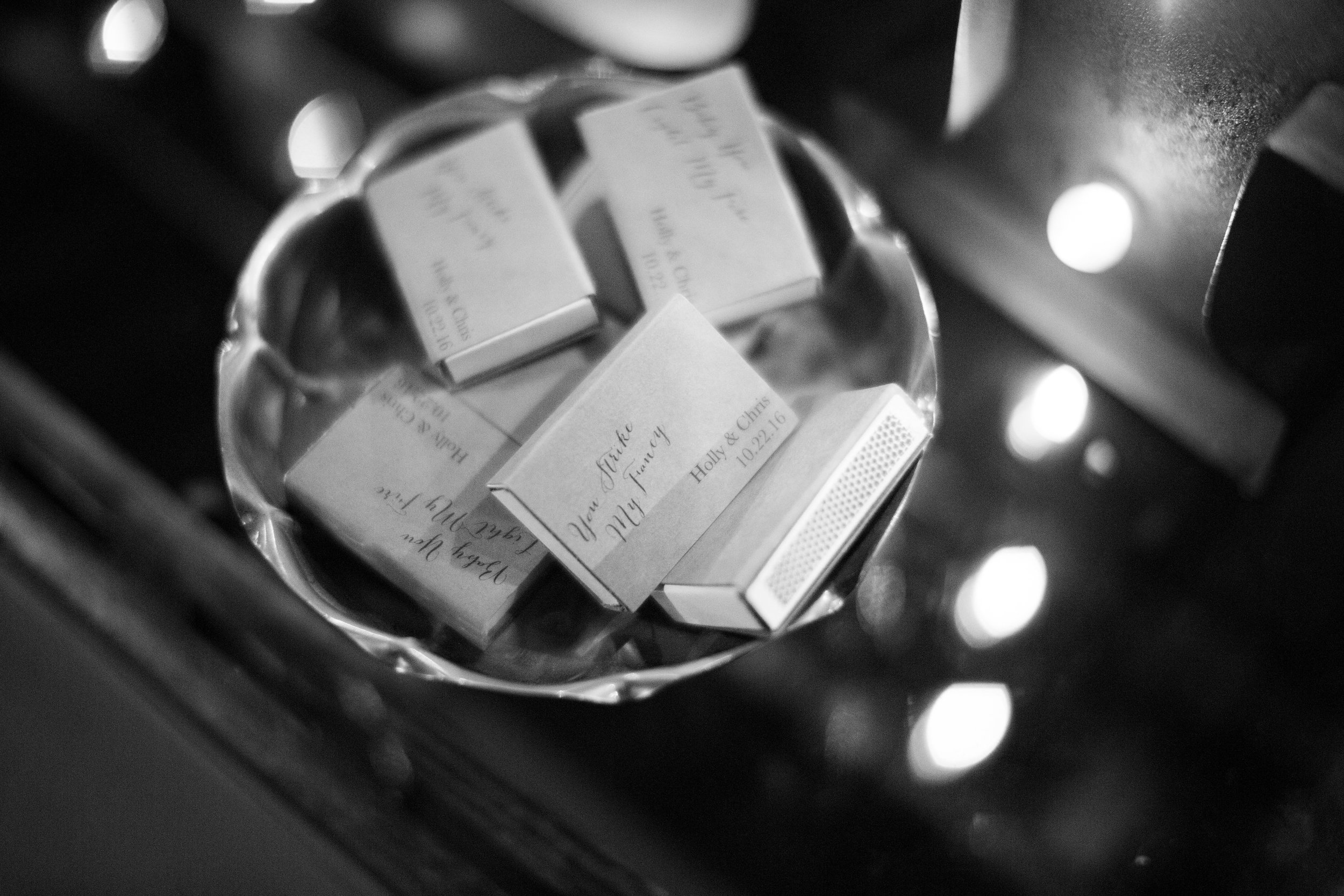In this elegant black and white photograph, a detailed silver bowl sits atop a shiny surface, likely a bar top, reflecting ambient light and adding a subtle glow to the scene. The bowl, adorned with ridges and a scalloped edge, contains several custom matchboxes. Each matchbox features a script that reads, "You strike my fancy," with "Holly and Chris, 10.22.16" inscribed below, suggesting these are wedding favors. The matchboxes are of an old-fashioned style, complete with a striking strip on the side. The image is artistically composed with a bokeh effect, causing most matchboxes to blur into the background, while a handful remain sharply in focus, highlighting the intricate details and giving the photograph a vintage, timeless quality.